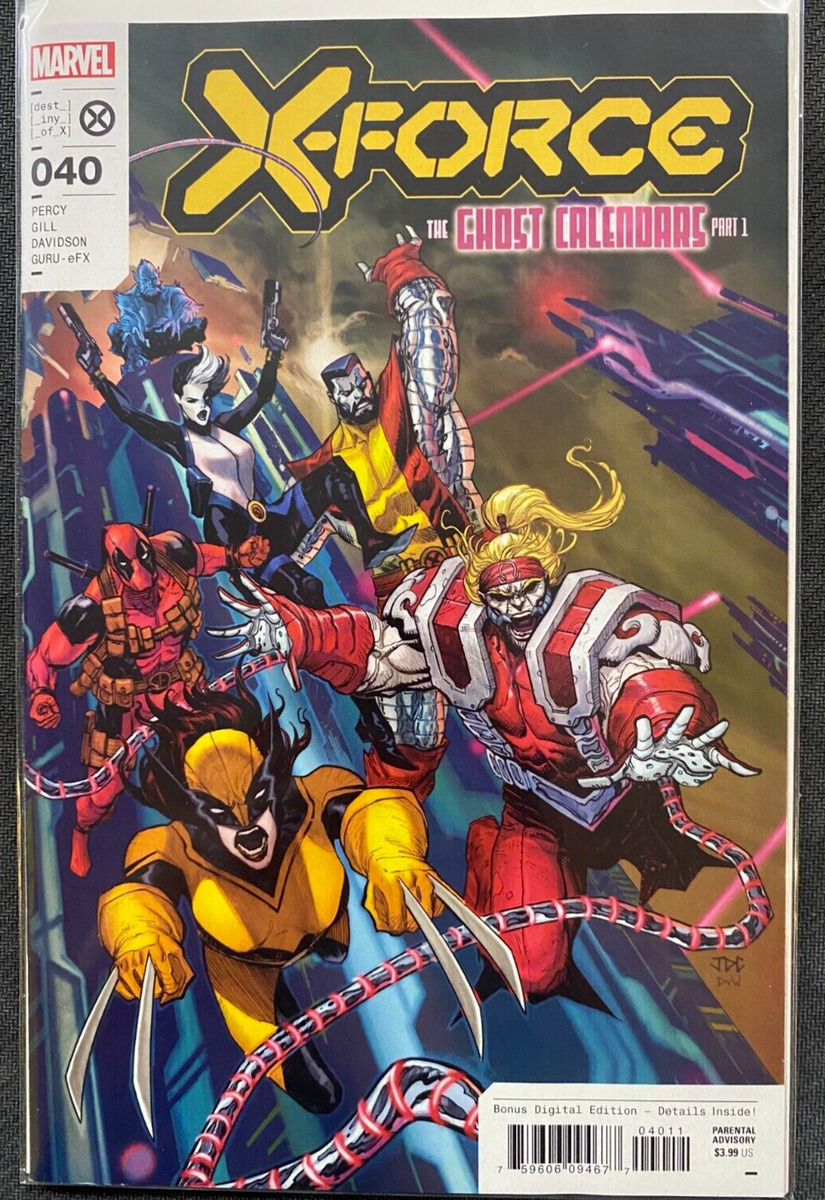The image is a detailed photograph of a Marvel comic book cover for "X-Force: The Ghost Calendars Part 1". The comic book title "X-Force" stands out at the top in bold, yellow geometric angular font, accented with a thick black border and a thinner yellow outer line. Below it, the subtitle "Ghost Calendars Part 1" appears in pink text with a white glow effect.

In the top left corner, a white rectangle contains the Marvel logo in white lettering against a red background, followed by additional lines of information. The comic is encased in plastic, confirming that it's a photograph rather than a scan, with its surface resting on a barely visible black cloth.

The cover features a vibrant assembly of superheroes. Starting from the lower left, there is a woman resembling Wolverine, lunging forward with metal claws extending from her knuckles, dressed in a yellow and black spandex suit. Next to her is Deadpool, depicted in his characteristic red and black jumpsuit festooned with brown pouches, also lunging at the viewer. To the right of Deadpool is Domino, clad in a black spandex jumpsuit with a white torso, her face white with a distinctive black shape over her left eye, holding guns in each hand. 

A prominent muscular man with a blonde ponytail and a monstrous white face stands to the right in red armor featuring large shoulder pads. Behind this figure is Colossus, a towering figure made of metal wearing a red jumpsuit with a yellow stripe down the center. The ensemble suggests a diverse and dynamic team of superheroes ready for action.

Additional elements include a barcode on the bottom right, and text indicating a "bonus digital edition" and "Parental Advisory," denoting the comic's price as $3.99 USD. The cover, wrapped in plastic, sits on a black cloth, confirming the physical nature of the comic in the photograph.